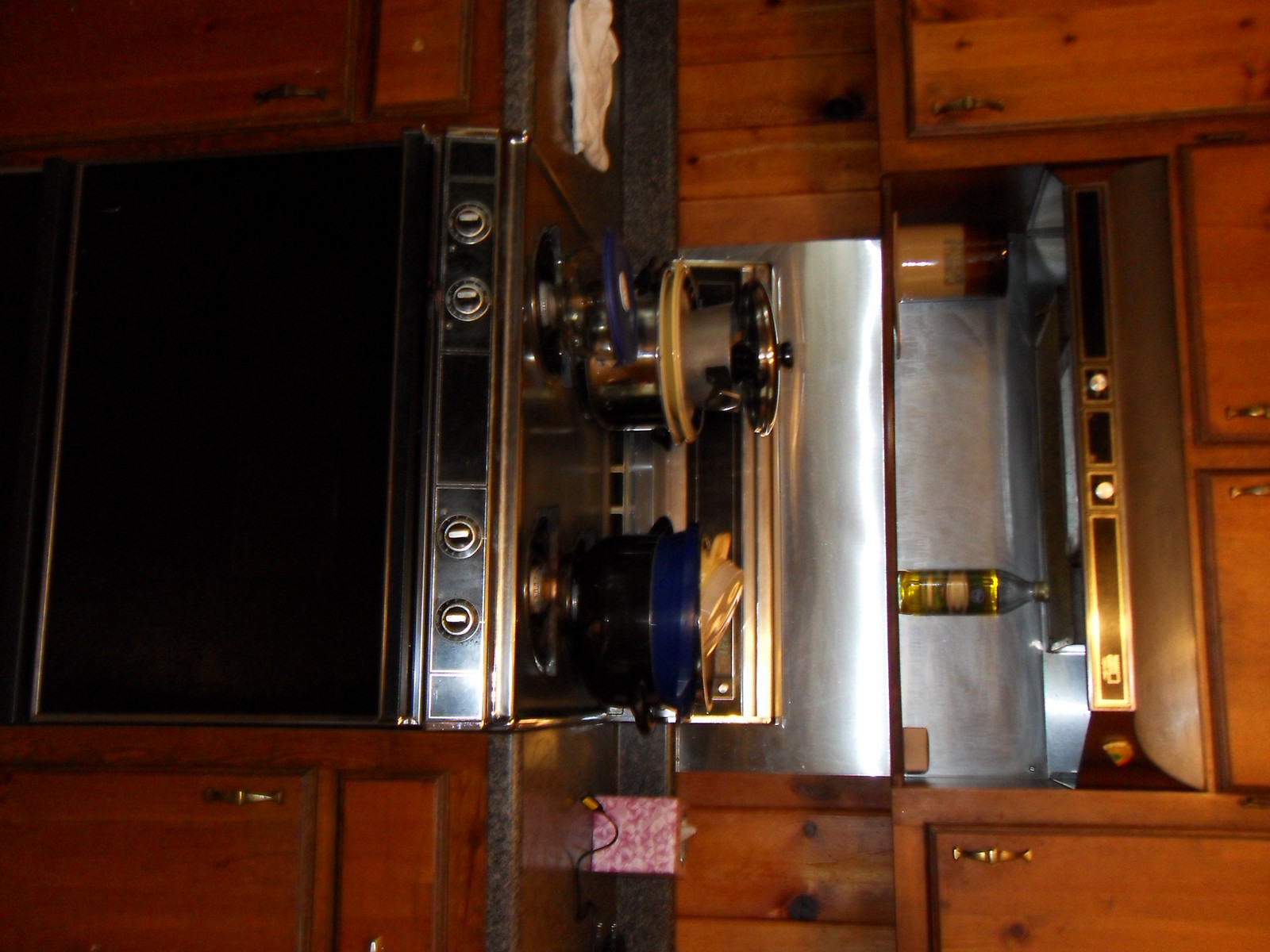The photo, slightly tilted to the right, reveals a rustic kitchen interior. The entire kitchen exudes a warm, wooden finish, with the exception of modern appliances. The countertops are a striking gray-black speckled granite, adding a touch of elegance. The stove, a classic black model with gold trimming and silvery-gold detailing on the handles and knobs, stands out against the predominantly wooden setting.

The gas stove, though currently off, hosts an array of kitchenware on its back burners. On the left burner, a silver pot is precariously stacked with a beige bowl, a smaller pot, and a lid. The right burner supports a black pot, a blue pot, and a beige container. Adjacent to this setup, a pink and white floral tissue box stands out, accompanied by a cord whose function is unclear.

Above the stove, the vent hood matches the stove's black and gold motif. A small shelf integrated into the hood features a large candle and a bottle of cooking oil, adding both practicality and charm to the kitchen's ambiance.

This beautifully detailed kitchen blend vintage and modern elements, creating a cozy, lived-in feel.